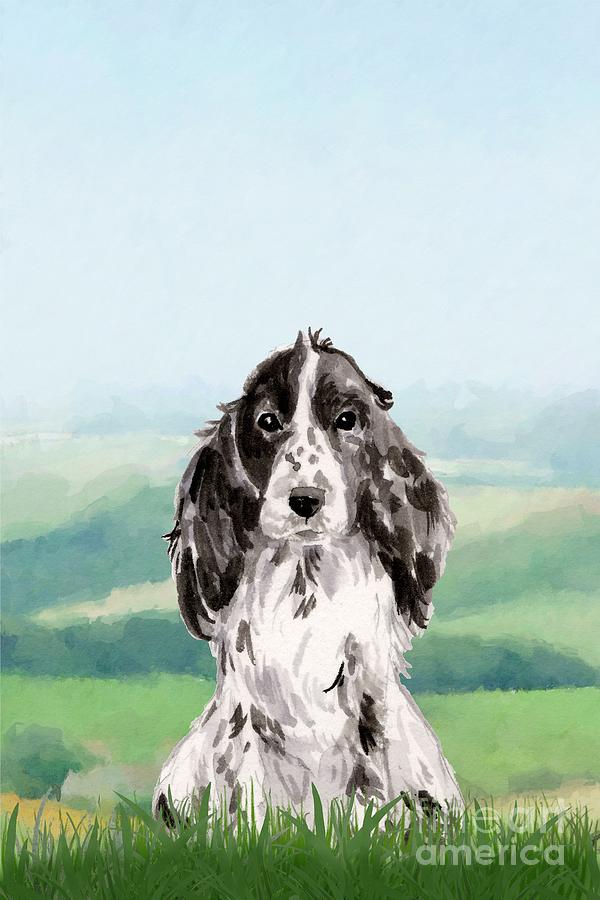This painting features a shaggy dog, likely a cocker spaniel, sitting in a field of green grass. The dog is primarily white with striking black ears and a black head, while a white section highlights its nose alongside a distinctive white stripe running down the center of its head. The lower part of its body is entirely white, blending seamlessly with its shaggy fur, obscuring its legs. The abstract background showcases a mix of green, depicting grassy areas and tree-covered hills that fade into gray, creating a sense of depth. The light blue sky covers the top half of the painting, enhancing the calm, pastoral scene. Notably, the painting bears the watermark "Fine Art America" in whitish lettering at the lower right corner, hinting at its artistic provenance. The medium used appears to be either acrylic or oil pastel, adding to the texture and vibrancy of the piece.